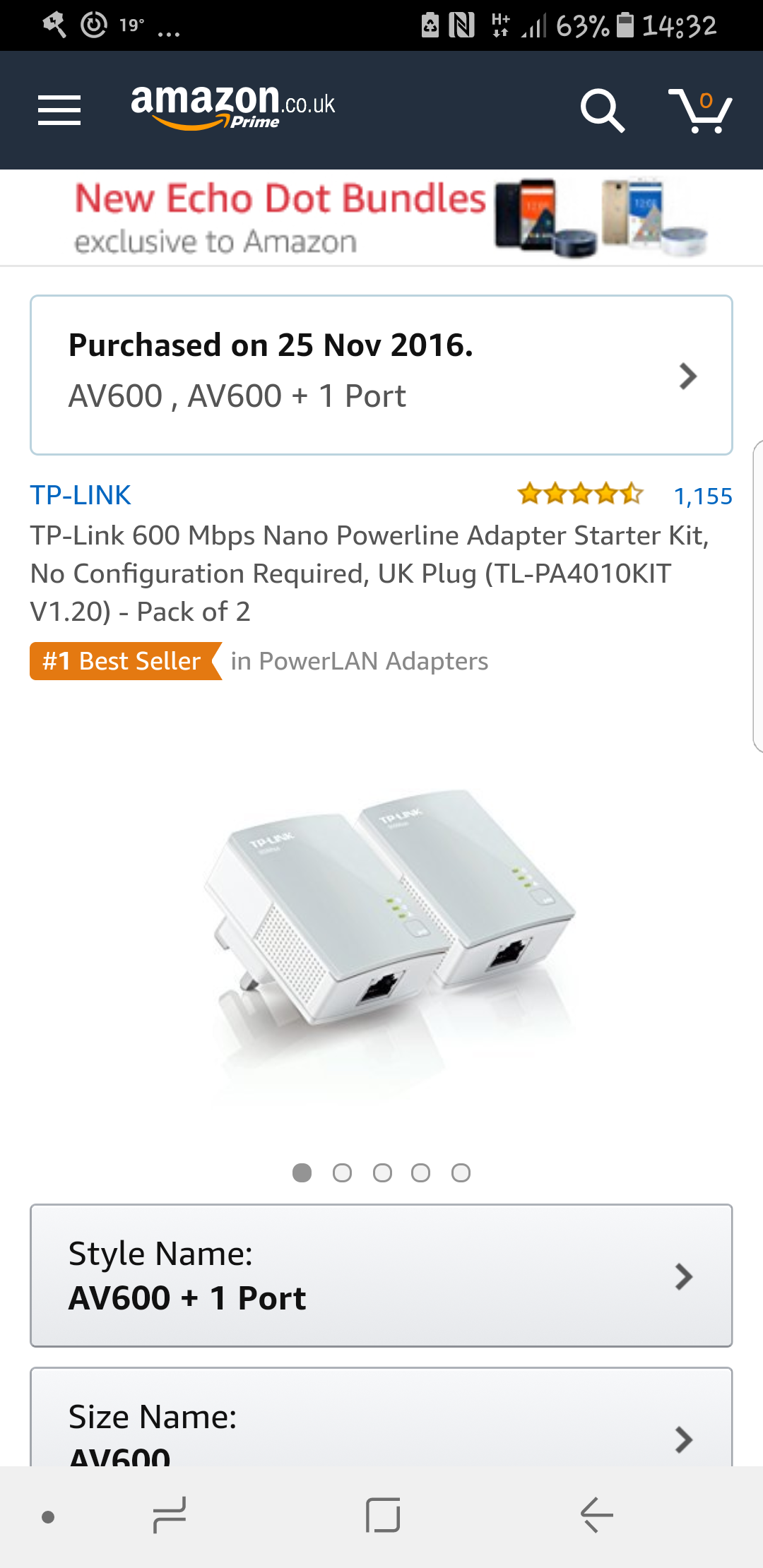This image depicts the Amazon UK website. The highlighted section showcases a prominent banner promoting "New Echo Dot Bundles Exclusive to Amazon Prime." Additionally, the page features a product listing for the "TP-Link AV600 Powerline Adapter Starter Kit" which is labeled as the "#1 Best Seller in Powerline Adapters." This particular product offers 600 megabytes per second of data transfer, requires no configuration, comes with a UK plug, and is sold in a pack of two. The adapters are white, thin, and square-shaped, featuring ridges on the side. The background of the image shows the plug and the bottom section where the connecting cord would be inserted. The style name of the product is "AV600 Plus One Port," and the size name is "AV600." The product was being promoted for purchase on November 25, 2016.